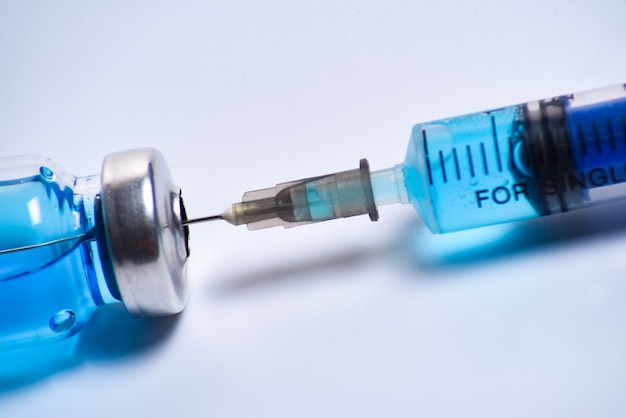The image is a close-up photograph of a syringe extracting blue liquid from a vial that is lying on its side. The vial, positioned on the left with its silver cap facing to the right, is partially covered with a blue exterior. The needle of the syringe is fully inserted into the vial, with the puncture point clearly visible. The syringe barrel, which features the label "4-S-I-N-G-L," likely indicating single use, shows the liquid being drawn in. The plunger is black with a dark blue column, creating a suction to pull the liquid into the syringe. The scene is set against a white table, under overhead lighting that casts soft shadows of the objects.